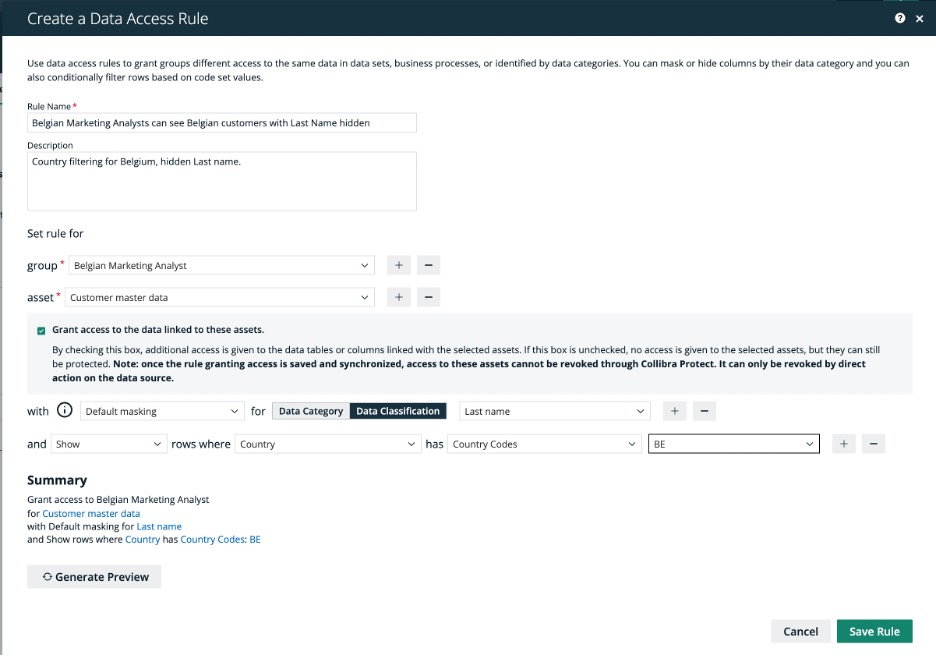The image depicts a webpage dedicated to creating a data access rule. Stretching across the top of the webpage is a horizontal black bar with the title "Create a Data Access Rule." Below the title, instructional text explains that data access rules allow for differentiated access to the same data within datasets by organizing business processes into various data categories. Users can opt to mask or hide data columns based on their categories, as well as conditionally filter rows by code set values.

The central part of the webpage features a form with several fields. A mandatory text box labeled "Rule Name" is filled with the entry "Belgian Marketing Analysis." The "Description" field is similarly populated with "Country filtering for Belgium, hidden last name."

Further down, there is a section titled "Set Rule For," containing two required fields marked with asterisks: "Group" and "Asset." These fields need to be completed by the user.

To the right, there is a light gray box bearing a check mark within a green square, accompanied by the instruction "Grant access to the data linked to these assets." Adjacent to this are fields for "With" and "And," set by default to "Meeting" and "Show" respectively.

At the bottom of the webpage, a summarized section is prominently marked with the header "Summary" in bold black text. This section reiterates the rule, stating "Grant access to Belgian Marketing Analysis." Beneath this summary, there's a button labeled "Generate Preview" in a gray box.

Numerous clickable blue links are embedded within the summary text, allowing for further navigation or actions related to the data access rule setup.